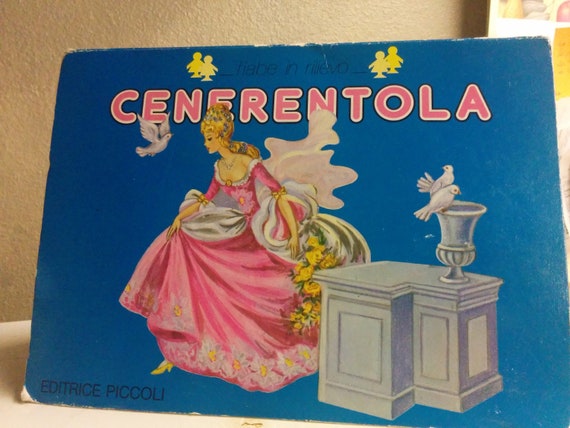The image is a rectangular card made of blue cardboard, with rough edges, likely resembling an advertisement or product packaging. Dominating the center, a blonde-haired woman is depicted in a very fancy pink ball gown with ample flowing skirts and intricate floral designs along the hem, accented by a white outline around the bodice. The dress is paired with golden high heels, and she holds a bouquet of yellow roses in her left hand. Her hair is styled mostly upward with some flowing down her back. A white dove is prominently positioned with its wings spread, seemingly fluttering in front of her. Above the woman, the word "CENERENTOLA" is written in rounded pink all-caps text. The top of the card features narrow black text on a blue background, which is somewhat hard to read and appears to be Italian, with words like "FIABE IN RILIEVO." Above this text are two pairs of yellow featureless figurines resembling children. On the far right of the card, there is an L-shaped gray stand with an urn or vase on top, and two white doves perched on its edge. The backdrop for the entire image is a consistent blue, providing a striking contrast to the vivid details of the characters and elements on the card.